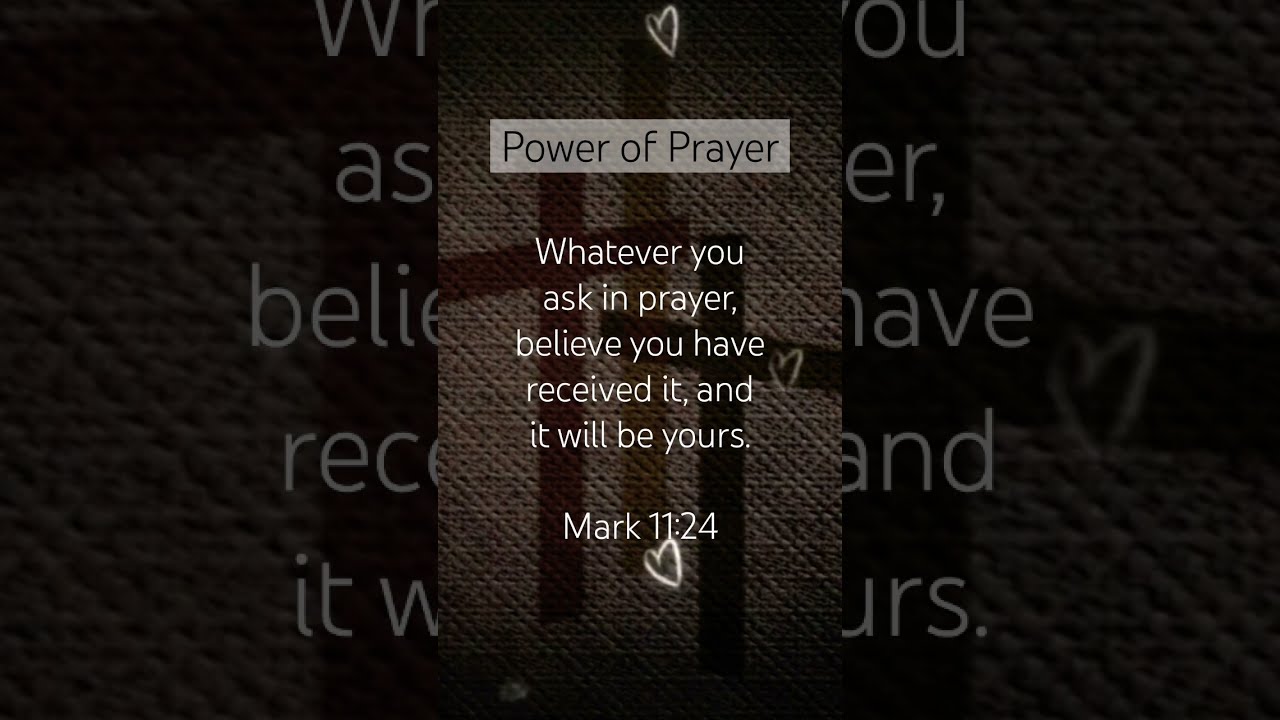The rectangular image, approximately six inches wide by three inches high, is a motivational, religious meme designed for mobile viewing. It features a central textured background resembling woven jute fabric. This fabric, with its thick weaving, is highlighted by three distinct vertical stripes: red on the left, gold in the center, and black on the right. Additionally, two diagonal stripes cross the image—a red one originating from the left and moving upward across the red and gold sections, and a green one coming from the right and stretching over the black and gold areas.

At the top of the image, a horizontal white rectangle with black text prominently displays the title: "Power of Prayer." Below this headline, in white text, is the inspirational quote from Mark 11:24: "Whatever you ask in prayer, believe you have received it, and it will be yours." This message is centered on the fabric background.

The image's design includes partial fragments of the central fabric motif on both the left and right sides, creating an enlarged, darker split effect that frames the main quote. Additionally, small details like a heart symbol at the bottom and several crosses in red, black, and brown hues enhance the religious theme.

Overall, the image is a visually detailed and symmetrical composition blending inspirational text with a rich, woven fabric design, underscored by subtle religious symbols and a motivational message.